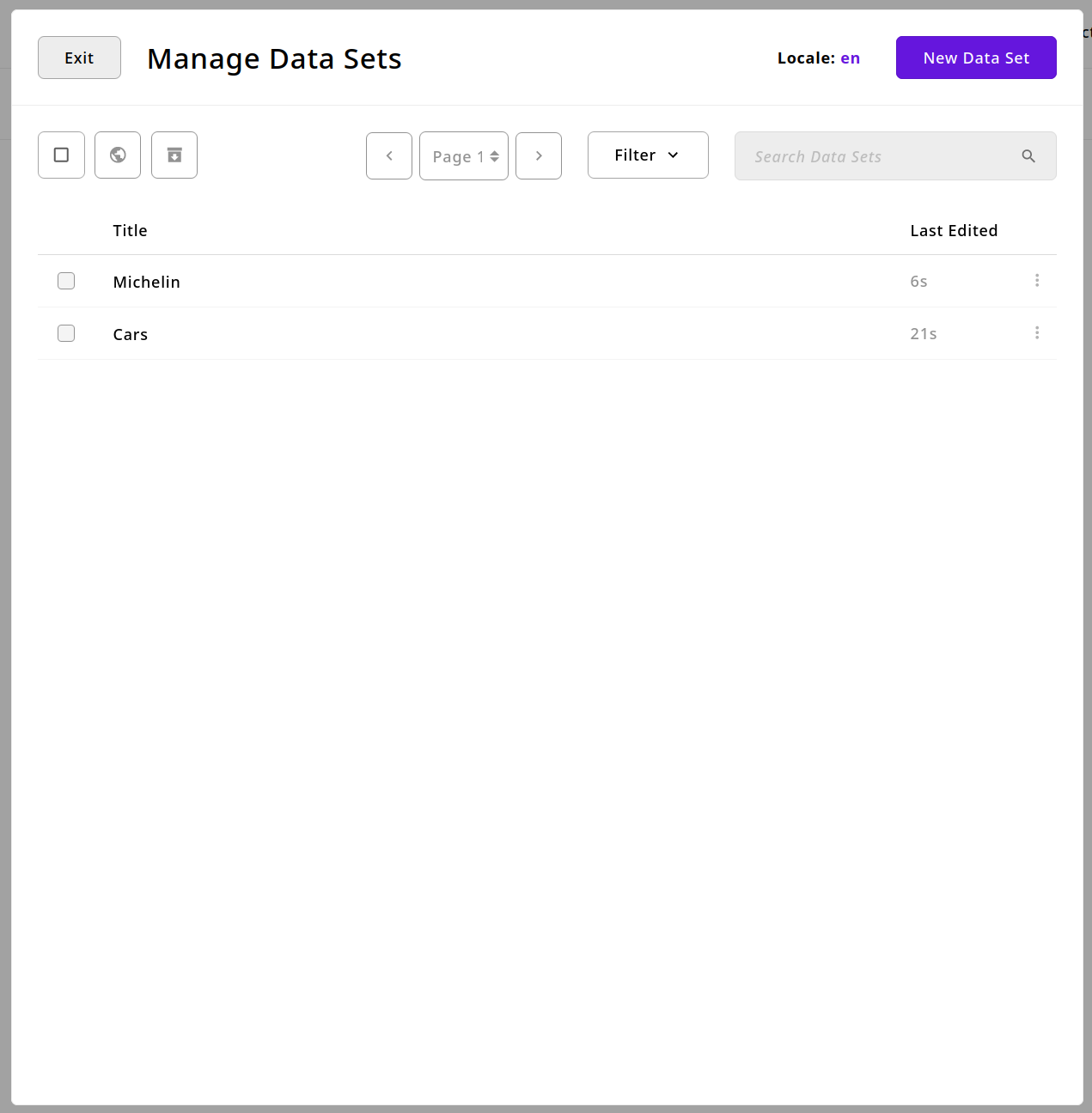The image depicts a user interface with a clean, structured design. The primary interface is a white block bordered by a double grey line. 

In the top left corner, there is a light grey button labeled "Exit." To the right of this button, prominently displayed in large font, is the title "Manage Data Sets." Moving to the far right, the word "Locale" is displayed in uppercase letters, followed by the status "On." In the very top right corner, a purple button with white text reads "New Data Set."

Directly below this header section is a row of functional buttons. The first small square button contains a square icon, the second has a circle icon, and the third features an indeterminate symbol. Next, there are navigation buttons including a left-facing arrow, a label "Page 1" with an up and down arrow for page navigation, and a right-facing arrow. Further along, there's a dropdown option under the label "Filter" and a dark grey search bar with the placeholder text "Search Data Sets" accompanied by a magnifying glass icon.

Beneath this functional row, the interface displays a table with two columns: "Title" on the left and "Last Edited" on the right, underlined by a thin grey line. The first row contains an empty checkbox next to the title "Michelin," which was last edited 6 seconds ago, along with three ellipsis dots indicating more options. The second row features another empty checkbox next to the title "Cars," last edited 21 seconds ago, also followed by three ellipsis dots.

Overall, the interface is designed for managing data sets with clear navigational tools, search functionality, and a list of data entries sorted by their last edited timestamps.